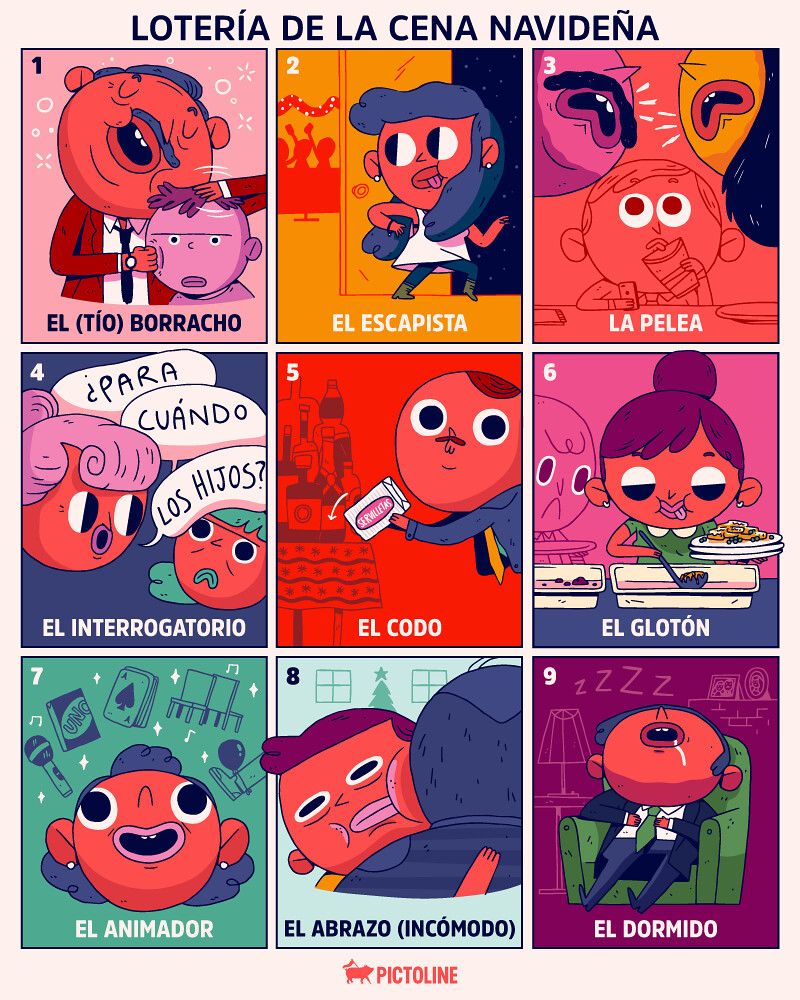This lively, colorful image, drawn in a cartoon style reminiscent of a comic strip, is entitled "Loteria de la Cena Navideña" at the top in bold Spanish text. The image is organized into nine squares arranged in three rows, each featuring a unique, whimsical scene painted in vibrant hues of orange, pink, red, and blue.

1. The first square, labeled "El Tio Baracho," depicts a man and a young boy, perhaps an inebriated uncle.
2. In the second square, "El Escapista," a woman tiptoes away, reminiscent of an escape artist sneaking out of a situation.
3. The third image, "La Pelea," shows a man and woman screaming at each other while a little boy sips from a juice cup, caught in the middle of the chaos.
4. "El Interrogatorio" appears in the fourth square, portraying a mother and son in a serious conversation.
5. The fifth illustration, "El Codo," is another character depiction, but its specifics are less clear from the descriptions.
6. The sixth square, titled "El Gloton," features someone indulgently eating.
7. "El Animador" in the seventh square likely shows an entertainer or someone hyping up the scene.
8. In the eighth square, "El Abrazo," there is an embrace, hinting at a moment of affection.
9. Lastly, "El Dormido," depicts a man who might be sleeping, crying, or drooling in a chair.

At the very bottom of the image, the word "Pictoline" is displayed, potentially the artist or the publisher's name.